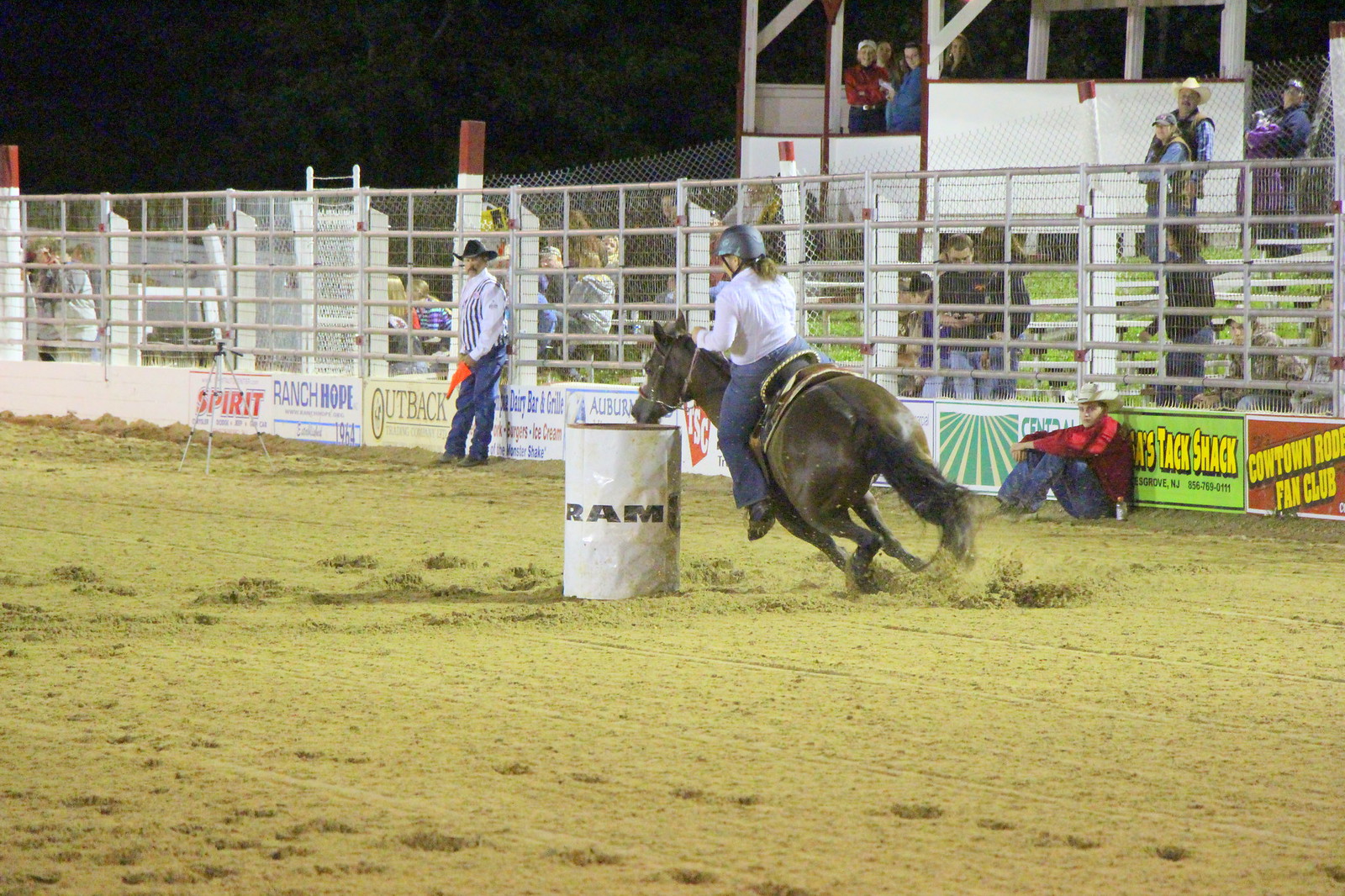The photograph captures a nighttime rodeo event with an intense barrel racing scene. At the center of the image is a white barrel labeled "Ram," placed on a corral covered with soft dirt, deeply imprinted by horse hooves. A dark brown horse with a black mane and tail is galloping around the barrel, moving from right to left. The rider, a female with Caucasian features and white-blonde hair, wears a black helmet, a long-sleeved white shirt, and blue jeans. 

In the background, a long, caged-in wall delineates the corral. To the right of the barrel inside the ring, a cowboy, dressed in a white hat, a long red-sleeved shirt, and blue jeans, sits on the ground. On the left, another cowboy stands near a tripod, wearing a black cowboy hat, a blue and white striped shirt, and blue jeans. 

Beyond the corral, stadium seating is partially visible, filled with spectators intently watching the action. The night sky is pitch black, and various advertisements for businesses line the fence, adding to the atmosphere of the event.